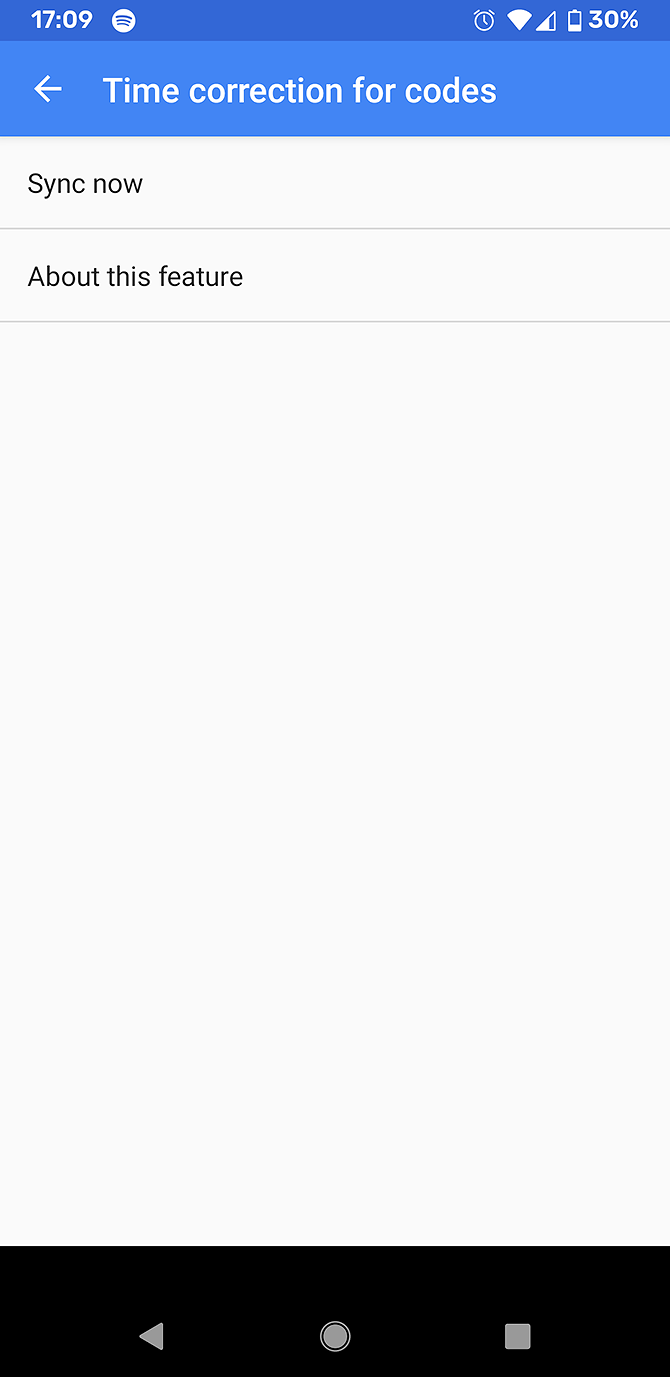This image is a screenshot taken from a mobile phone. In the upper left corner, a blue banner displays the time as 17:09, accompanied by a small white circle to its right. On the upper right corner, icons indicate an active alarm clock, full Wi-Fi signal, and a battery level at 30%. Below the banner, white text reads "Time correction for codes," with a white arrow pointing left. 

Against a white background, dark gray text states "Sync now," separated from the subsequent text by a light gray horizontal line. Further below, another section in dark gray text reads "About this feature," also separated by a light gray line. The bottom portion of the screen is largely blank, dominated by a large white area. At the very bottom, a black bar features three navigation icons: a left-pointing triangle, a circle, and a white square.